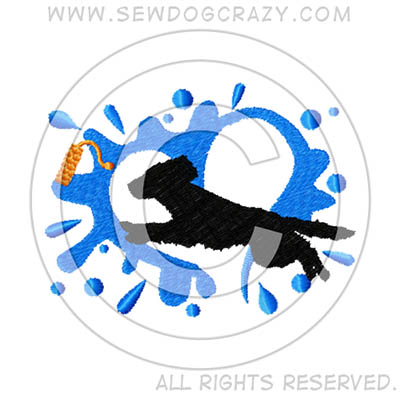The image is a hand-drawn logo for a website, prominently featuring the URL www.cdogcrazy.com at the top. The central design showcases a simplistic black dog in mid-jump, with the movement creating vivid blue splotches that resemble splashing water. These splotches are arranged to form a subtle heart shape in white behind the dog, symbolizing passion and care. An intricate watermark of the letter "C" within a circle is embedded across the design, blending seamlessly but remaining visible. To the far left, there is a depiction of a thread, hinting at a sewing theme. The lower right corner of the image is marked with "All Rights Reserved," reinforcing the logo's protected status.